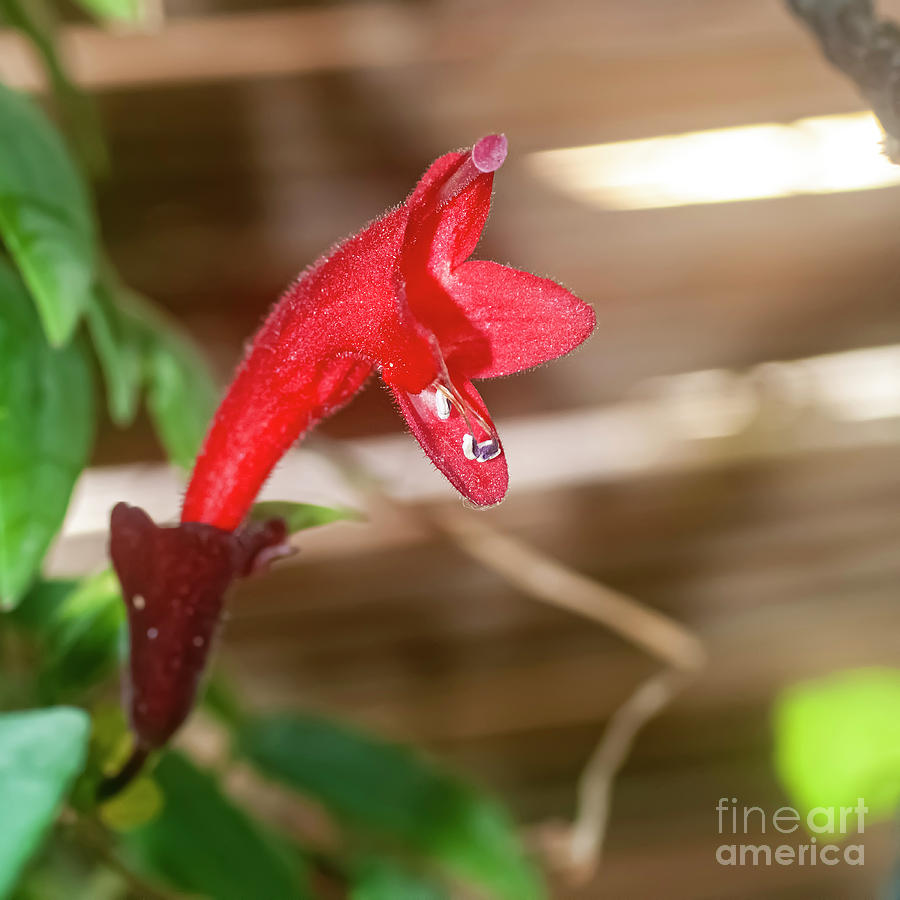This striking photograph by Fine Arts America features a vivid red flower prominently displayed in the center. The flower, with its spiny petals adorned with delicate water droplets, rises from a pot with green leaves visible in the background. Exhibiting a blend of natural beauty and fine detail, the background is beautifully blurred to emphasize this vibrant bloom, which has a unique elongated structure where it meets its green stem. The backdrop includes earthy tones of brown and hints of wood and dirt, adding to the rustic charm of the scene. Subtle branding is present with the Fine Arts America logo in the bottom corner, discreetly integrated to maintain the visual appeal of the artwork.